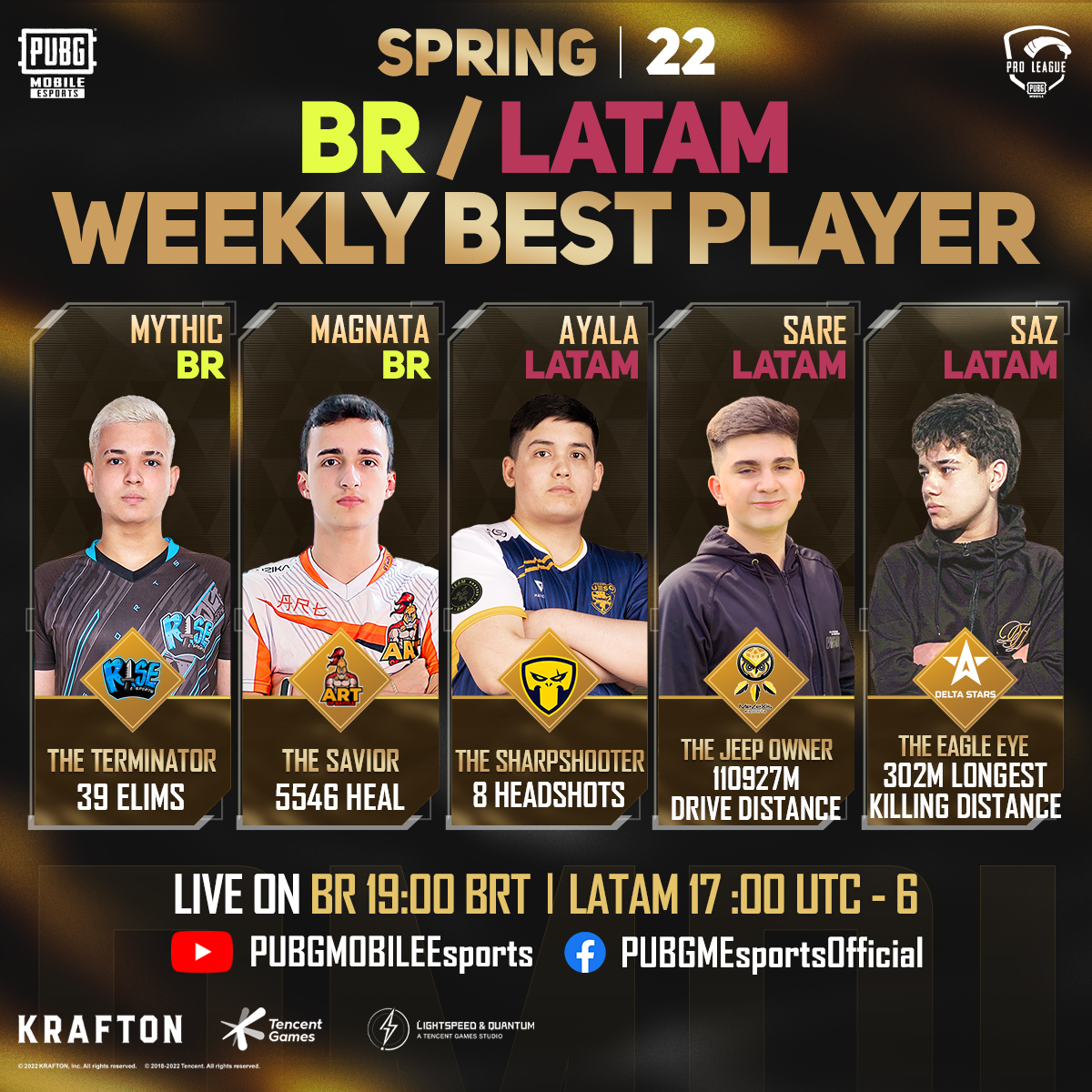The poster is an advertisement for a video game event. At the top, it prominently displays "Spring '22" with "BR" in yellow letters and a tan slash followed by "LATAM" in red letters. Below, in gold letters, it reads "Weekly Best Player." Five male players are showcased from left to right, each with their in-game name, title, and specific achievements. 

- The first player, Mythic BR, labeled "The Terminator," has 39 eliminations.
- The second player, Vagenta BR, known as "The Savior," has achieved 5546 heals.
- The third player, Ayala LATAM, called "The Sharpshooter," has scored eight headshots.
- The fourth player, Sare LATAM, titled "The Jeep Owner," has a drive distance totaling 110927 meters.
- The fifth player, Saz LATAM, identified as "The Eagle Eye," boasts the longest killing distance of 302 meters.

Below the players, the poster declares "Live on BR 19:00 BRT / LATAM 17:00 UTC-6," indicating the broadcast times. It also features the PUBG Mobile eSports logo and mentions the official social media channels on YouTube and Facebook under "PUBGME Sports Official." In the bottom left corner, the poster credits Crafton and Tencent Games, with a logo for Lightspeed and Quantum featuring a lightning bolt. There's small, unreadable text at the very bottom. The background is black with various texts in colors like yellow, red, gold, and white, creating a vibrant and informative promotional image.